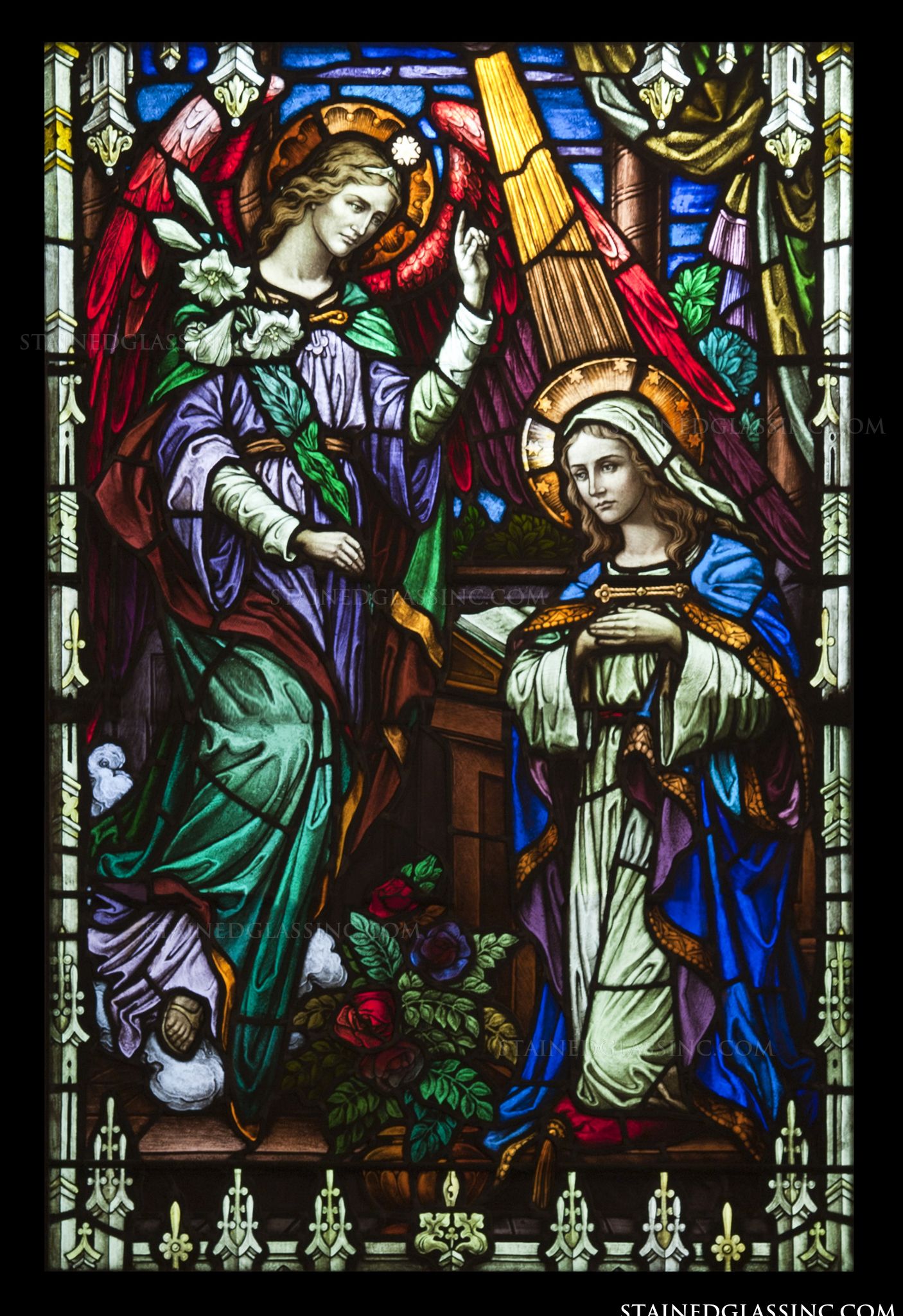The stained glass window depicts a profoundly ecclesiastical and Christian-themed scene featuring two prominent figures set against a colorful and intricate backdrop. On the right, the Virgin Mary is depicted with a serene and graceful demeanor, adorned in a blue shroud over a white dress, complemented by a white veil and a golden halo embellished with stars. She kneels with hands folded in front of her as she receives what appears to be divine instruction. At the top right, delicate white flowers rest on her shoulder, adding to her sanctified presence.

Opposite her, on the left side of the window, stands an angel, likely the Angel Gabriel, distinguished by his radiant red wings and halo. He is characterized by light brown hair and is dressed in a purple shroud over a green robe. Gabriel holds a bunch of lilies and appears to be imparting a message to the Virgin Mary. The backdrop is a harmonious blend of vivid colors including dark blue, red, and green, with elements such as green shrubs, a Bible on a pedestal, and both decorative and ecclesiastical motifs. The scene is framed with a decorative yellowish-white border, detailed with the text "StainedGlassInc.com," which also appears as a watermark in the center of the image.

Overall, the stained glass artwork is rich with religious symbolism, vibrant in its use of color, and detailed in depictions, capturing a poignant moment of divine communication.